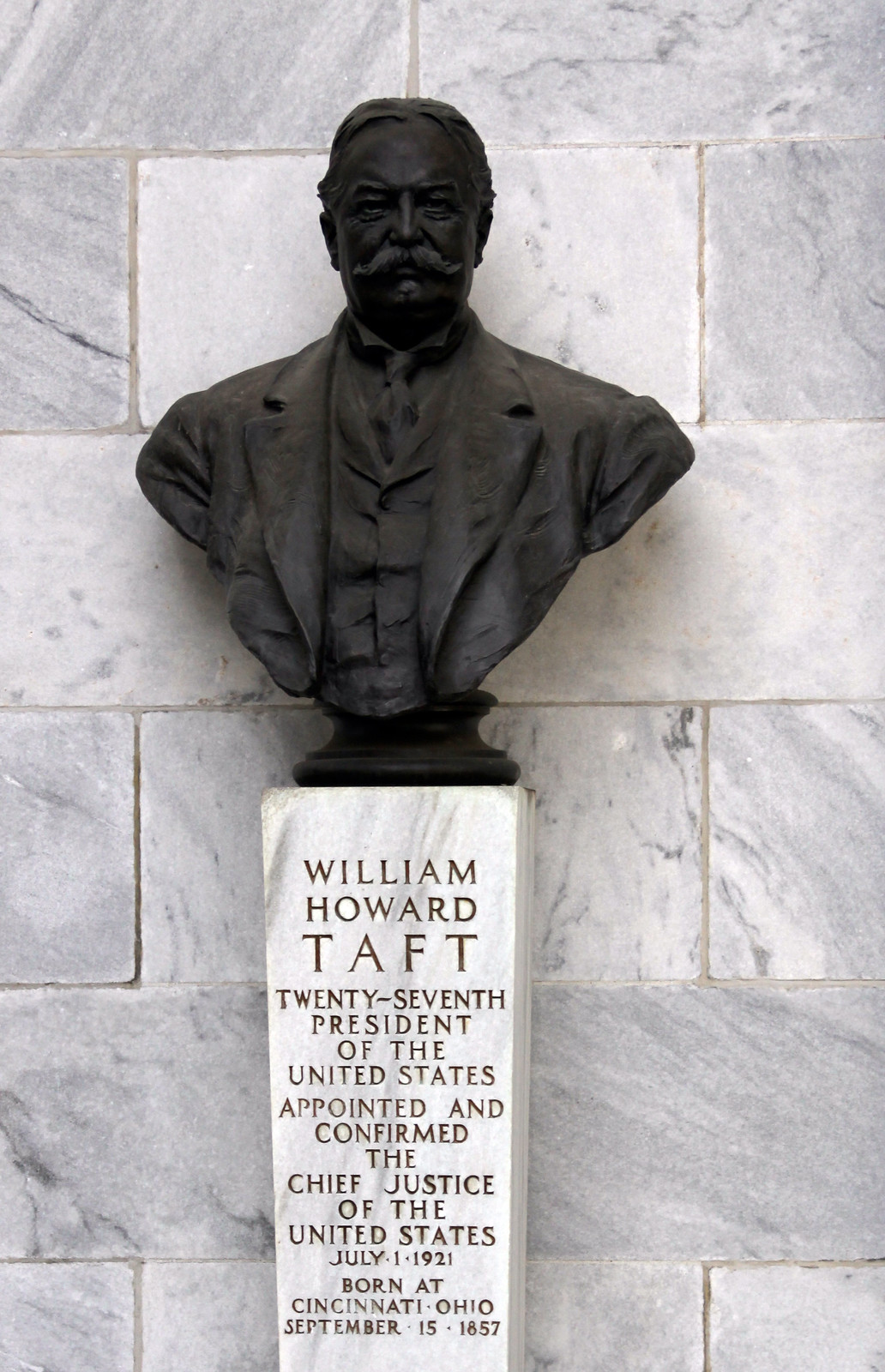The image features a black stone bust of William Howard Taft, prominently positioned at the center. The bust realistically captures Taft's head and shoulders, which taper down into a V shape at the chest. Taft's distinctive facial features include a thick mustache, a sliver of facial hair beneath his bottom lip, and slightly wavy hair. He is depicted wearing a business suit complete with a coat, vest, and tie. The bust sits atop a marble pedestal that bears the inscription: "William Howard Taft, 27th President of the United States, appointed and confirmed as Chief Justice of the United States, July 1, 1921, born at Cincinnati, Ohio, September 15, 1857." The pedestal is set against a textured background made up of offset individual gray and white marble slabs, suggesting a solemn and monumental setting that could be either indoors or outdoors.